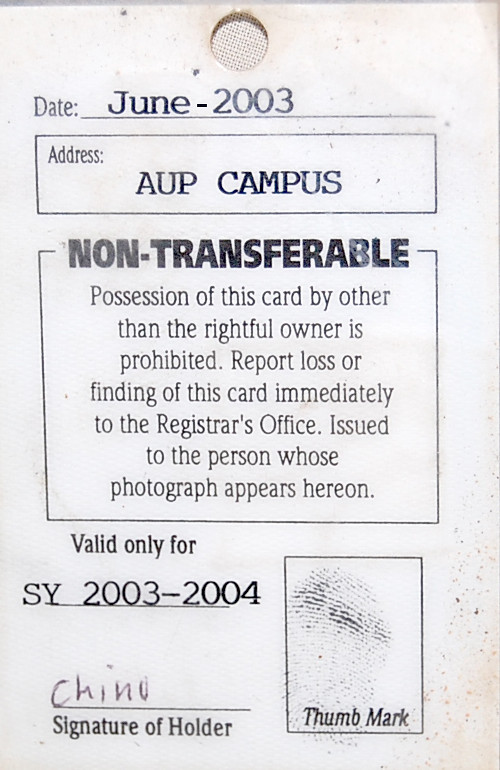This is a detailed photograph of an old, discolored, rectangular identification card, taller than it is wide, with a punched hole at the top center, presumably for attaching a string or lanyard. Behind the hole, a light tan woven fabric is visible. The card, originally white, now shows signs of age with gray, brown, and yellow dirt imprints along the edges. 

At the top left, below the hole, the card reads "Date: June 2003" in dark black ink. Below this, it displays "Address: AUP Campus" within a rectangular box. 

Prominently featured in bold print is the notice: "Non-transferable. Possession of this card by other than the rightful owner is prohibited. Report loss or finding of this card immediately to the registrar's office. Issued to the person whose photograph appears herein." This paragraph is bordered.

Further down, to the left, the card states "Valid only for SY 2003-2004." Beneath this line, "Chino" is handwritten in ink above the preprinted "Signature of holder." On the lower right, a rectangular box contains a small, faded black ink thumbprint, labeled "Thumb mark."